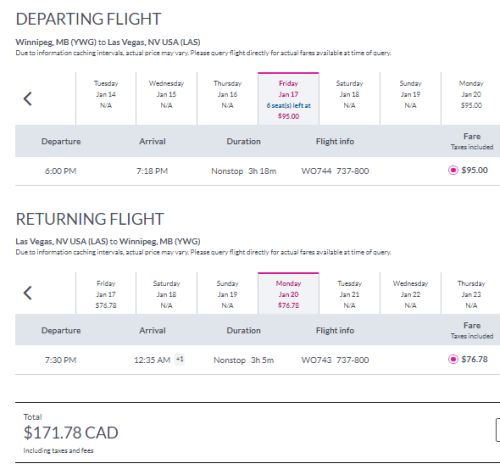Screenshot of Delta Flight Booking Webpage:

The image displays a nearly completed flight booking webpage from Delta Airlines. It confirms a round-trip itinerary from Winnipeg, Manitoba (YWG) to Las Vegas, Nevada (LAS). The departure flight is on Friday, January 17th, with six seats available at $95. The flight details include a departure time of 6:00 p.m. with an arrival time of 7:18 p.m., indicating a nonstop flight lasting 3 hours and 20 minutes. The flight number is W0744737-B00. 

The return flight is scheduled for Monday, January 20th, with a fare of $76.75. It departs at 7:30 p.m. and arrives at 12:35 a.m. the next day, showing a +1 symbol to indicate the next day arrival. This return flight also is nonstop, with a duration of 3 hours and 5 minutes, and follows the same flight number.

The total fare for both flights, including taxes and fees, amounts to $171.78 CAD (Canadian Dollars). This comprehensive price breakdown is displayed prior to final checkout.